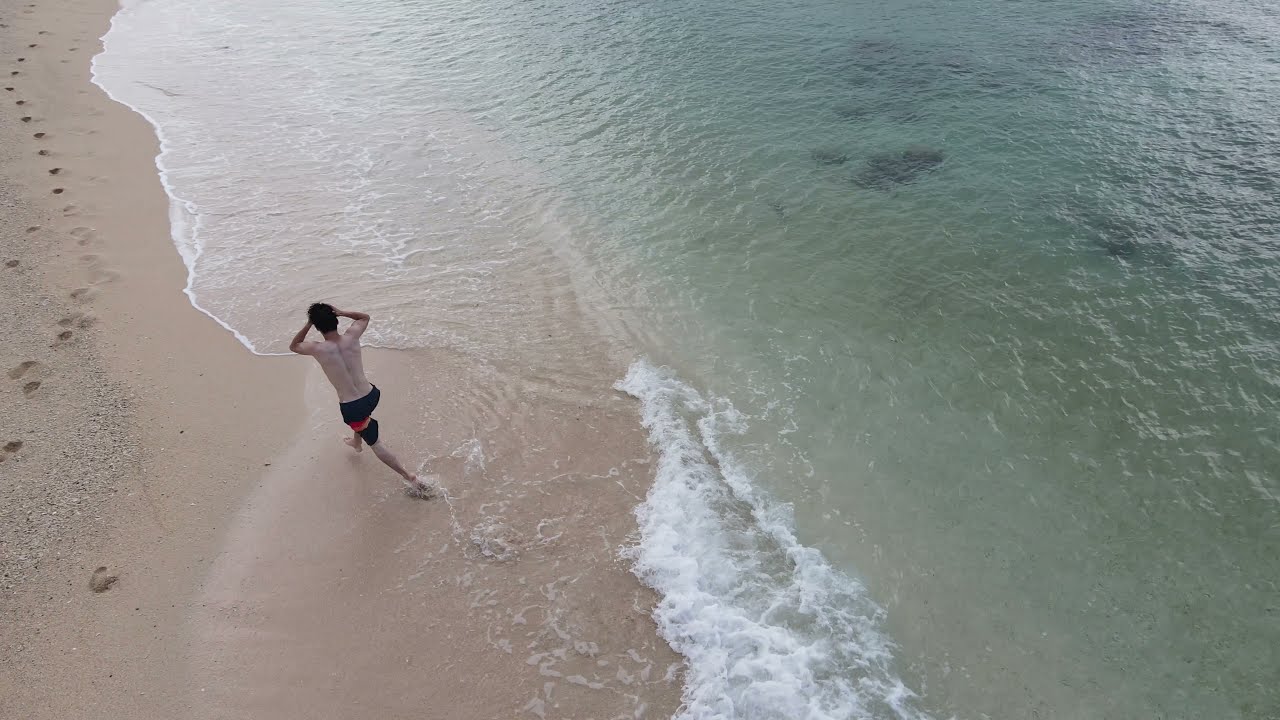A vibrant aerial photograph captures a tranquil coastal scene in stunning detail. Taken from a drone at a beach, the image features a young, shirtless man with black hair and both hands resting on his head. He is walking diagonally towards the upper left corner, partially immersed in the shallow, clear waters. His black and red swimming trunks stand out against the sandy beige shore to his left. Visible in the sand are round footprints trailing away into the distance. The gentle waves create a white, bubbly foam as they meet the shore at the bottom of the image. To the right, the water transitions from a clear see-through to a light aqua, dotted with dark spots that could be algae or seaweed, revealing rocks beneath the surface. The water appears calm with subtle ripples, occupying about two-thirds of the frame, and contrasts beautifully with the beach's serenity. This photograph, with its realistic and representational style, offers a serene snapshot of a beachside moment.